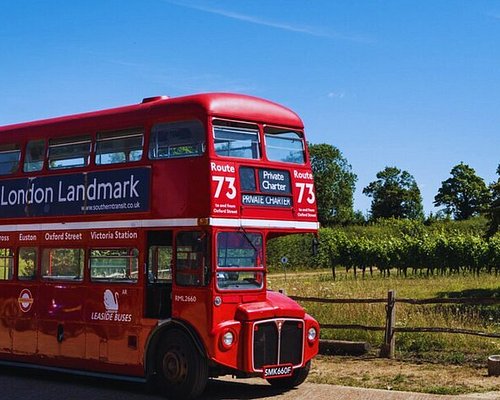The image captures a vibrant, red double-decker bus, distinctly marked with "Private Charter," traveling through a picturesque countryside setting. The bus, identified as Route 73, prominently displays "London Landmark" across its upper side, alongside a detailed image of a swan. On its lower side, the bus lists key destinations including Oxford Street, Victoria Station, and Leaside Buses. The scene is set on a sunny day with a clear blue sky, presenting no visible clouds except perhaps a jet stream. The bus is viewed from its right side and slightly from the front, positioned before a rustic, unpainted wooden fence that lines a grassy field dotted with small trees and shrubs. In the distance, a dense gathering of various types of plant life completes the pastoral backdrop. The road the bus is on appears paved, yet there are no visible passengers or driver inside this quintessentially British icon.